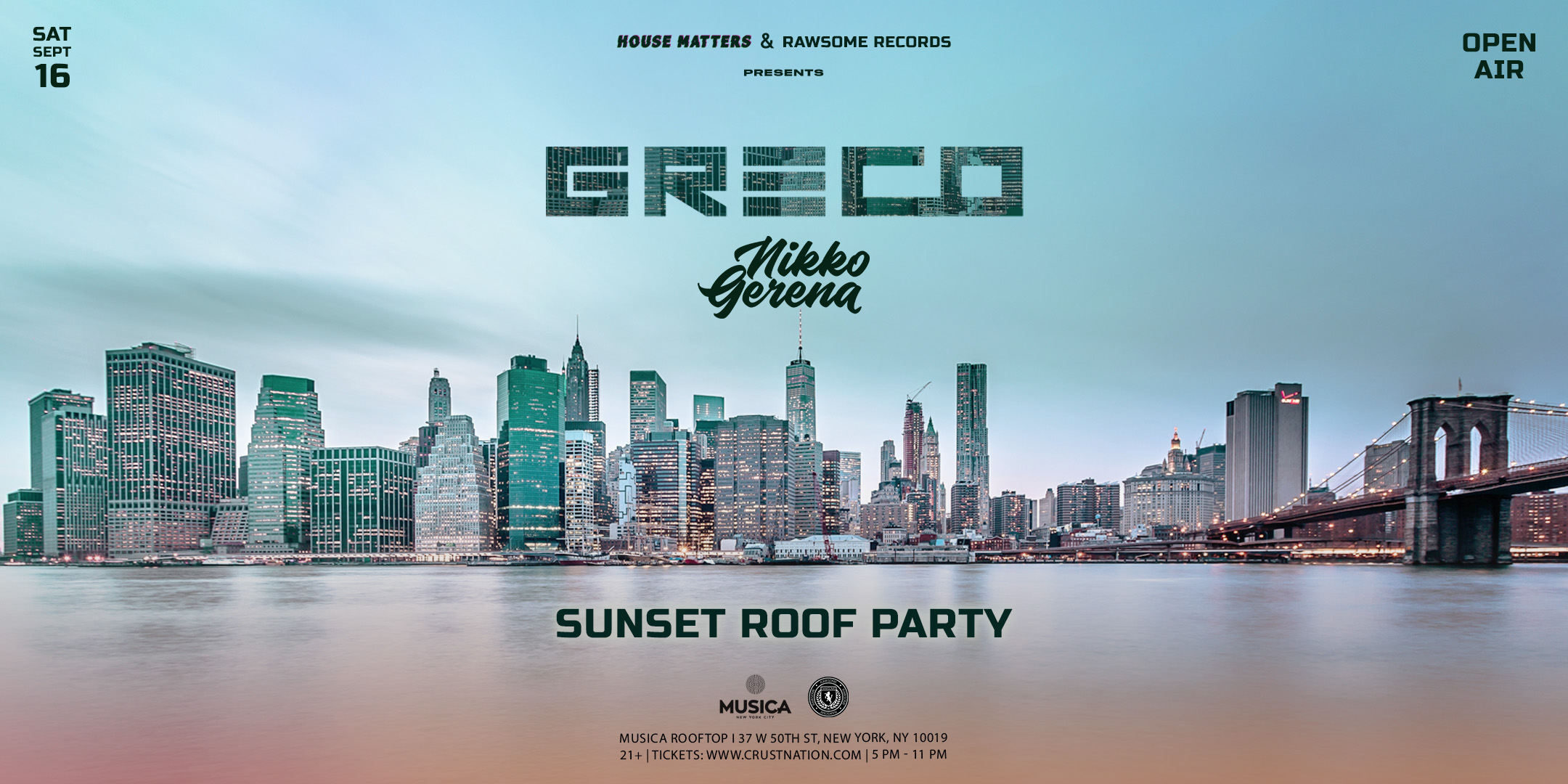The image is an advertisement for an event, featuring a blend of photograph and text. At the top, in black writing, it states "Center House Matters and Rossum Records presents Greco, Nico Jirina." The sky above is light blue and slightly hazy. Below, a cityscape in blue, gray, and purple tones stretches across with a skyline featuring tall buildings with yellow lights, especially on the left where they appear teal-tinted, transitioning to gray on the right. A distinctive bridge spans over water on the right side, with a big stone structure in the middle and ropes attached. The water at the bottom is shiny, reflecting grayish and brownish hues. In the center-left, it says "Sat Sept 16," and on the upper right corner, "open air."

Lower down, the image includes details about the event: "Sunset Roof Party" hosted at Musica rooftop, located at 37 West 50th Street, New York, NY 10019. It also notes that the event is for 21+ attendees, with tickets available at www.crustnation.com, and the event running from 5 p.m. to 11 p.m. A black circle logo in the lower section and icons of bottles add to the design elements. The Greco logo is stylized to resemble building shapes, intricate and integrated into the urban theme of the image.